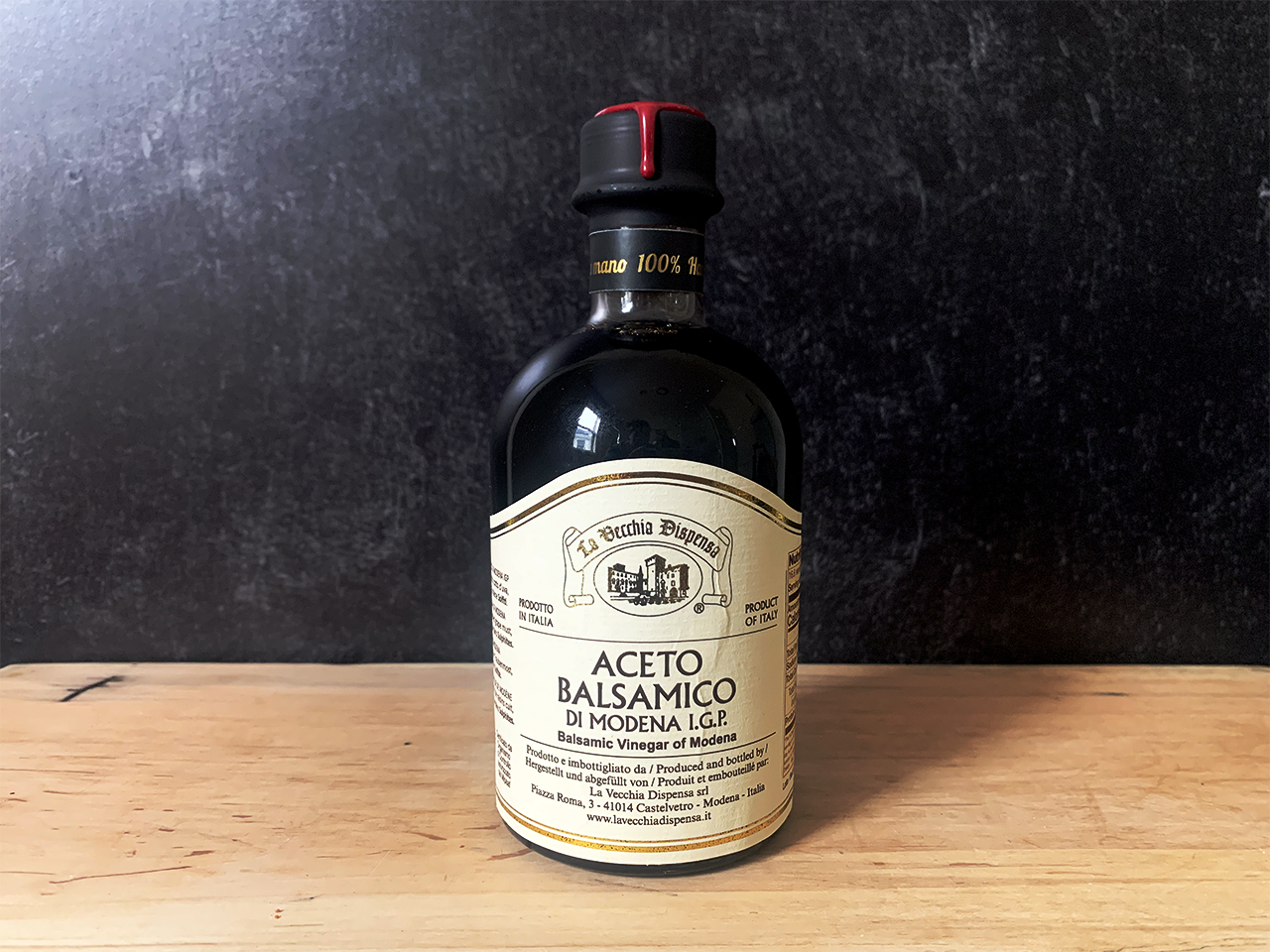The image showcases a high-end bottle of Balsamic Vinegar of Modena, prominently labeled "Aceto Balsamico di Modena." The dark, almost black bottle sits on a light-colored wooden surface, possibly a cutting board or a worn, light-blue scratched table. The bottle is distinguished by its elegant design, featuring a red wax seal drizzling down from the top and a black band with gold text around the neck. The label is a light tan with gold accents and black text, displaying the brand "La Bocchia Dispenza" and emphasizing its authenticity with "100% Balsamic Vinegar." The scene is set against a dark, textured background that appears to be either dark marble or painted concrete, enhancing the bottle’s sophisticated appearance. This product is unmistakably marked as a product of Italy, steeped in traditional craftsmanship.